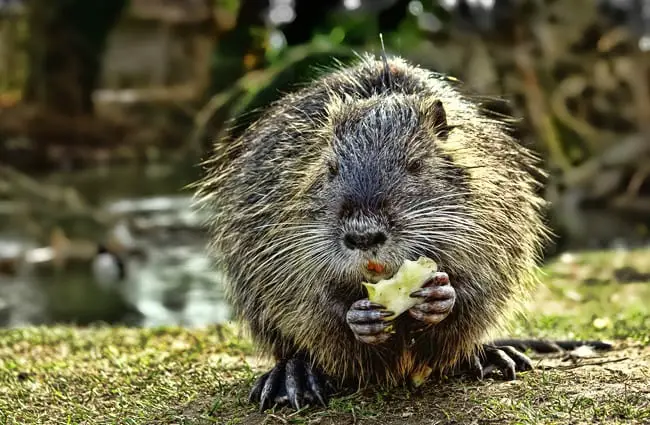In this detailed photograph, a brown and white beaver is prominently featured, slightly right of center, and facing the camera. The beaver is hunched over, occupying a patch of short, light green grass, and is holding a green apple slice in its front paws. Its gray face, accented by long white whiskers and a black nose, is focused as it eats. The beaver’s large, clawed hind feet are visible, as well as its distinctive flat tail extending behind it.

The background depicts a small creek to the left, with larger trees along its opposite shore. Additionally, there are some blurry gray bushes and green leaves visible in the right-hand side of the image. The animal's serene demeanor suggests it is contentedly enjoying its meal in this natural setting.